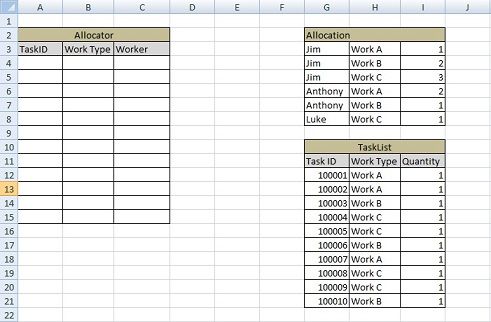The image features a detailed table set against a light gray background. The table is organized with columns labeled from A to J at the top in black text. There are light gray horizontal lines running across the table for alignment.

### Central Section (A to C, Rows 2 to 15):
- A large black-outlined box spans columns A to C from rows 2 to 15.
- Inside this box, row 13 is highlighted in yellow.
- The text inside the box reads "Allocator" in black against a beige background.
- Directly beneath row 3, the box lists "Task ID," "Work Type," and "Worker."
- Vertical and horizontal lines from rows 2 through 15 are outlined in black ink.

### Right Section (G to I, Rows 2 to 8 and 10 to 21):
- A similar black-outlined box spans columns G to I from rows 2 to 8.
- This box is labeled "Allocation by 2."
  - Rows 3 through 8 detail assignments:
    - Jim: Work A, No. 1
    - Jim: Work B, No. 2
    - Jim: Work C, No. 3
    - Anthony: Work A, No. 2
    - Anthony: Work B, No. 1
    - Luke: Work C, No. 1
- A second box spans columns G to I from rows 10 to 21.
- This box is labeled "Task List" in row 10.
  - Rows 11 through 21 list:
    - 10001: Work A, No. 1
    - 10002: Work A, No. 1
    - 10003: Work B, No. 1
    - 10004: Work C, No. 1
    - 10005: Work C, No. 1
    - 10006: Work B, No. 1
    - 10007: Work A, No. 1
    - 10008: Work C, No. 1
    - 10009: Work C, No. 1
    - 10010: Work B, No. 1

The overall layout is meticulously organized, allowing clear visualization of tasks and allocations across different sections of the chart.